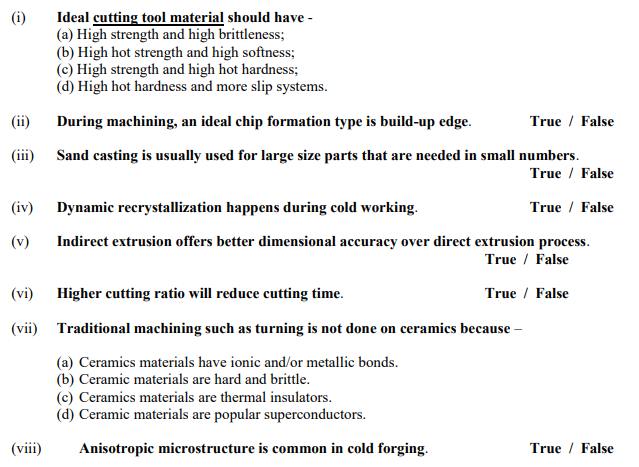The image displays a text-based quiz divided into eight sections, labeled with Roman numerals. Each section contains a question relating to material science or engineering principles. The first question, in bold, asks what the ideal properties for a cutting tool material are, offering four multiple-choice answers: A) high strength and high brittleness, B) high hot strength and high softness, C) high strength and high hot hardness, or D) high hot hardness and more slip systems. The second question prompts whether the ideal chip formation type during machining is "built-up edge," to be answered with true or false. The third question states that sand casting is generally used for large parts needed in small quantities and asks for a true or false response. The fourth question inquires if dynamic recrystallization occurs during cold working, with a true or false choice. The fifth question asks about the dimensional accuracy of indirect extrusion compared to the direct process, also answered true or false. The sixth question states that a higher cutting ratio will reduce cutting time and seeks confirmation through a true or false answer. The seventh question is another multiple-choice query, asking why traditional machining such as turning is not performed on ceramics, providing four options: A) ceramics have ionic or metallic bonds, B) ceramics are hard and brittle, C) ceramics are thermal insulators, or D) ceramics are popular superconductors. The final question addresses whether an anisotropic microstructure is common in cold forging, to be answered true or false.